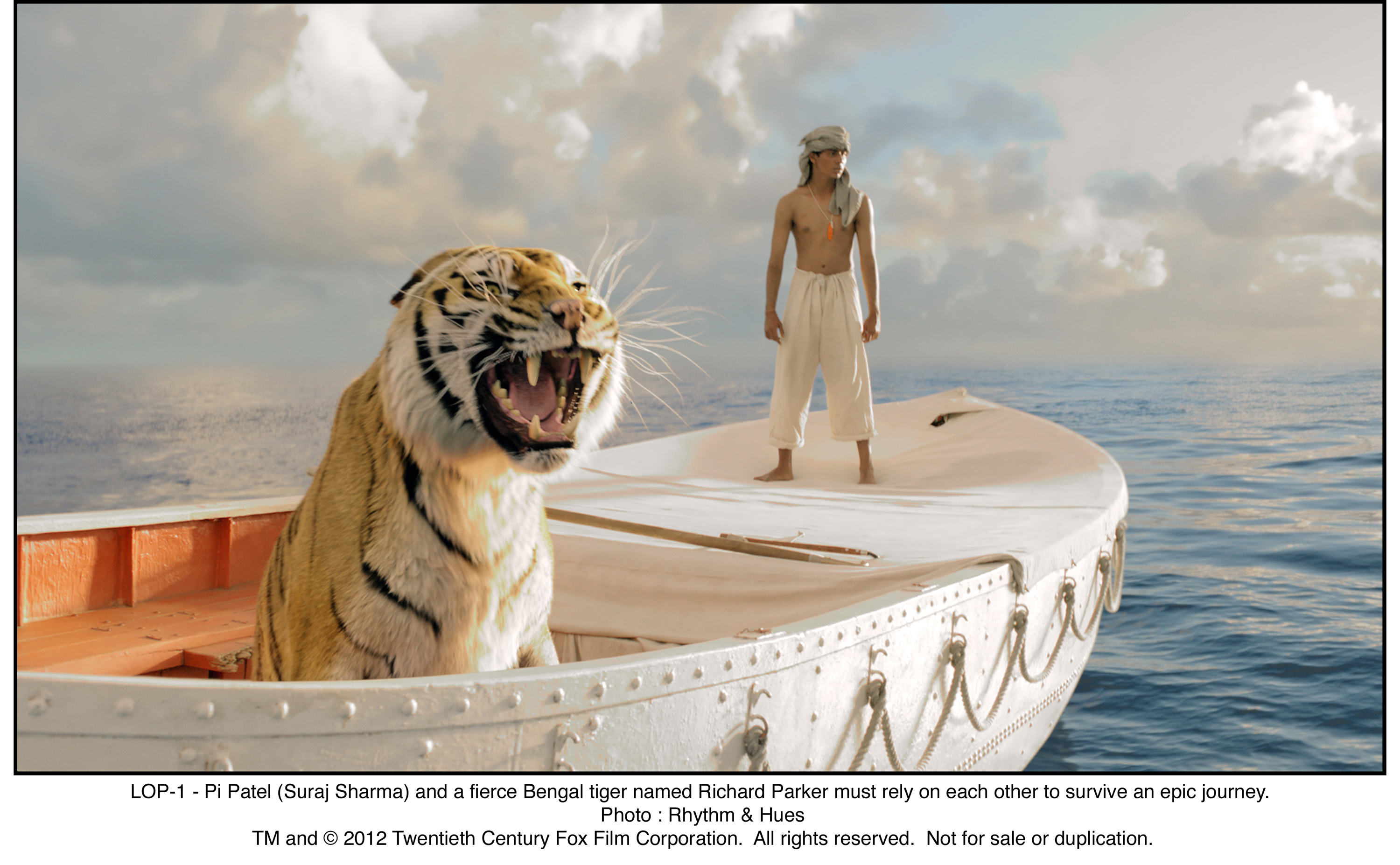The image is a promotional photograph with a thin black border, capturing a dramatic scene set in the middle of the ocean. At the center is a white wooden boat angled at approximately 75 degrees from the bottom left to the top right. The boat's interior is orange. Above the horizon, the sky is depicted with scattered white clouds. On the prow of the boat stands a shirtless man, smaller in scale as if photoshopped, wearing white pants and a towel or rag draped over his head, hanging over his left shoulder. An orange necklace dangles on his chest. Closer to the foreground in the boat sits a fierce Bengal tiger, mouth open in a growl. The bottom of the image features text in black that identifies the scene as part of a movie: "LOP1, P. Patel, Siraj Sharma, and a fierce Bengal tiger named Richard Parker must rely on each other to survive an epic journey." The photograph is credited to Rhythm and Hues and marked with "TM and 2012 20th Century Fox Film Corporation, all rights reserved, not for sale or duplication."